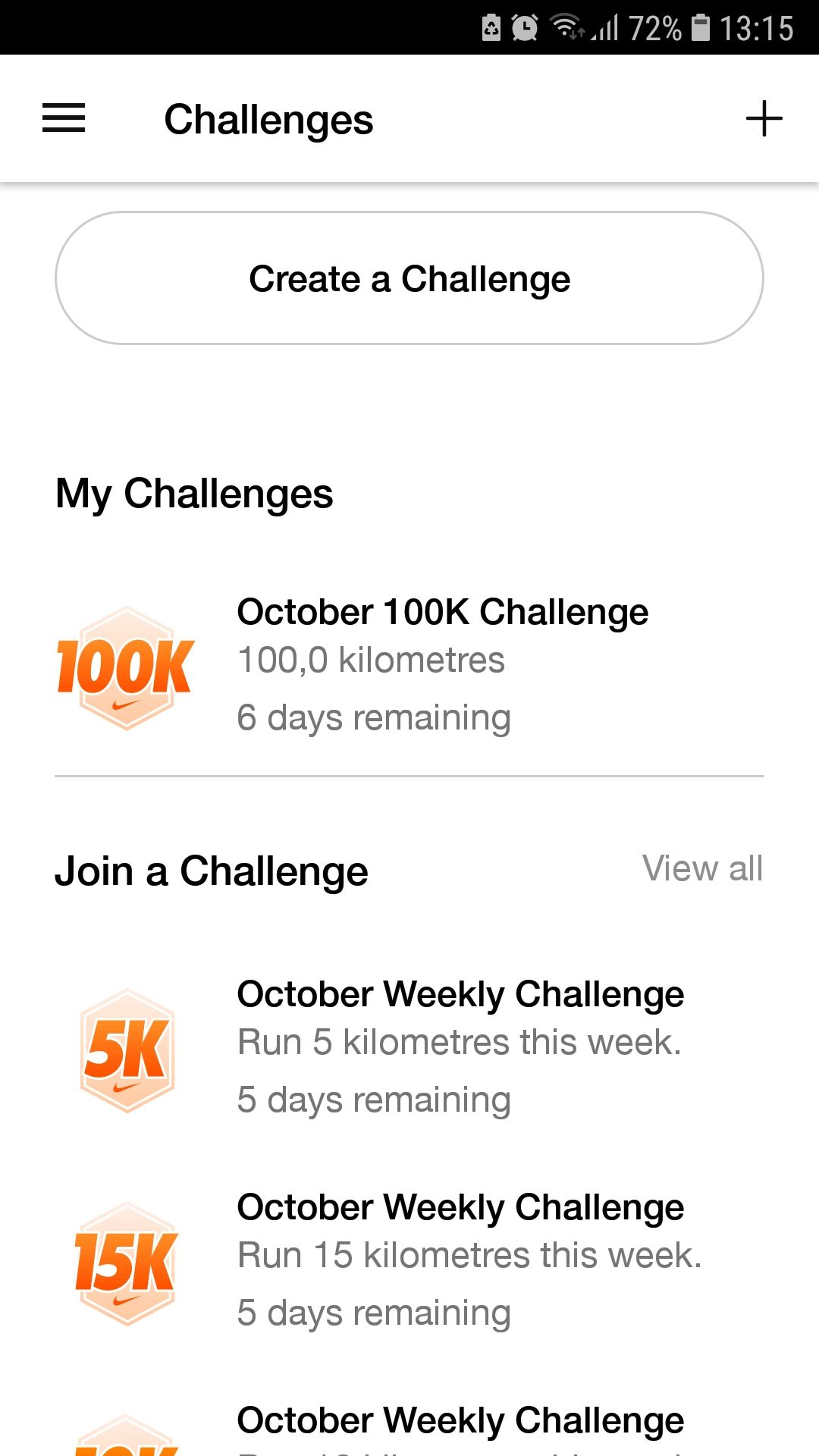The image displays a digital interface layout with several visual elements and textual information.

- At the top of the screen, there's a black rectangle. On the right-hand side of this rectangle, a series of symbols is visible:
  - A partially discernible icon that resembles a rectangle with an arrow inside it.
  - A clock icon.
  - A Wi-Fi symbol.
  - A signal strength indicator with bars growing taller from left to right, displaying 72%.
  - A battery icon showing 3:15.

Below this, three black lines are stacked vertically. The text "Challenges" appears next to these lines on the left, and there is a plus sign on the right. Beneath this section is a thin gray line.

Following that, a light gray, bulging rectangle contains the text "Create a Challenge." Below it, the header "My Challenges" is displayed. 

Further down, a light orange shape is marked with "100K" in orange text, accompanied by a small orange checkmark. The text reads:
- "October 100K Challenge"
- "100.0 kilometers"
- "Six days remaining."

Below this section, there is another thin gray line and the text "Join a Challenge," with "View All" on the right.

The next segment includes:
- A light orange symbol labeled "5K" in brighter orange with an orange checkmark underneath. The text reads:
  - "October Weekly Challenge"
  - "Run five kilometers this week"
  - "Five days remaining."

Following this is another light orange symbol marked "15K" with an orange checkmark underneath. The text reads:
- "October Weekly Challenge"
- "Run fifteen kilometers this week"
- "Five days remaining."

At the bottom, the top of an orange shape and partial text of another challenge can be seen. The visible text indicates:
- "October Weekly Challenge."